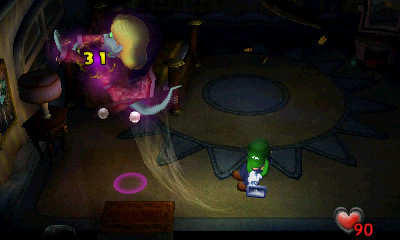This image showcases a scene from a video game set inside a room with a distinctive floor design. At the center of the floor is a blue circle encased within a tan circle, which is further surrounded by blue triangles forming an intricate pattern. In the room, there is a small table adorned with a lamp and lampshade. Seated on the floor is a character who appears to be Luigi from the Super Mario Bros. franchise. Adding a touch of fantasy to the scene, a character with blonde hair and dressed in pink is seen hovering in the air. At the bottom of the screen, an interface element displays a heart symbol accompanied by the number '90', suggesting this might be indicative of health or another in-game resource.